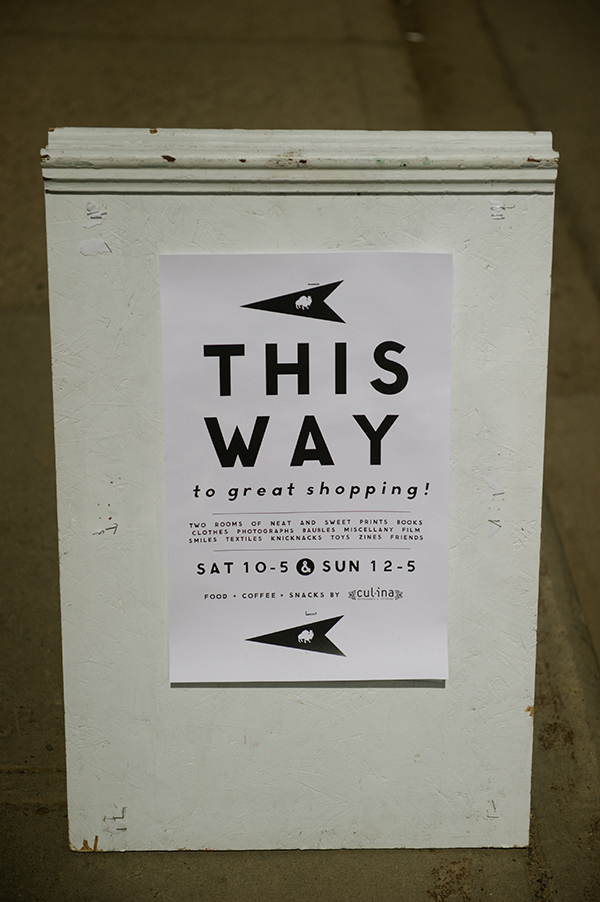The image is a color photograph of a white piece of paper taped to an upright, white-painted, rectangular wooden stand, placed in a blurry, grayish, stone-like background. The paper, adorned with black text, prominently features a leftward-pointing arrow at the top, directing viewers to "This Way to Great Shopping" in bold capital letters and italicized lowercase letters. Below this, additional details are listed in smaller print: "Two Rooms of Neat and Sweet Prints, Books, Clothing, Photographs, Baubles, Miscellany, Films, Smiles, Textiles, Knickknacks, Toys, Zines, and Friends." The sign also includes the activity times, "Saturday 10 to 5 and Sunday 12 to 5," and mentions available refreshments: "Food, Coffee, Snacks by Culina." Another leftward arrow with a buffalo-like design is placed at the bottom. The stand appears to be set on a rough, stone or cement surface, which creates an out-of-focus background, enhancing the visibility of the sign’s important and inviting message.